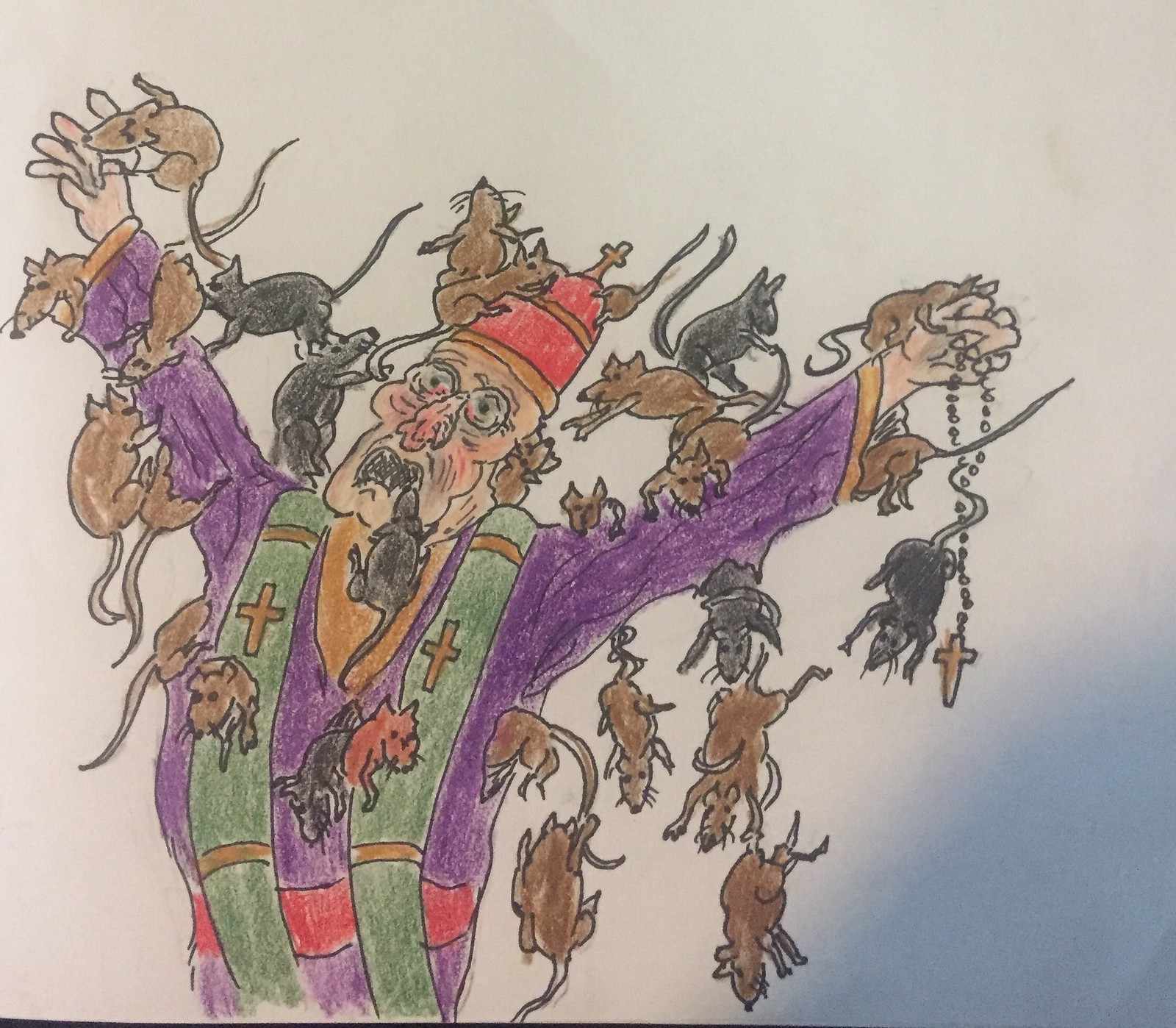A crayon drawing on a white background features a distressed-looking man standing prominently on the left side. He is depicted from the front with raised arms that extend outward at an angle. The man sports a long face with wide, white eyes and a downturned mouth, creating an expression of distress. He wears a red hat adorned with a horizontal brown line and a brown cross on top. His attire includes a purple robe and a distinctive green scarf around his neck, which is decorated with brown horizontal lines near the shoulders, brown crosses in the center, and additional brown lines towards the bottom.

Crawling all over him are black and brown mice, adding to the chaotic and unsettling nature of the scene. From his right hand dangles a chain composed of small black circles, ending in a brown cross. In the lower right-hand corner of the drawing, there is a patch of blue, providing a contrasting background to the rest of the illustration.